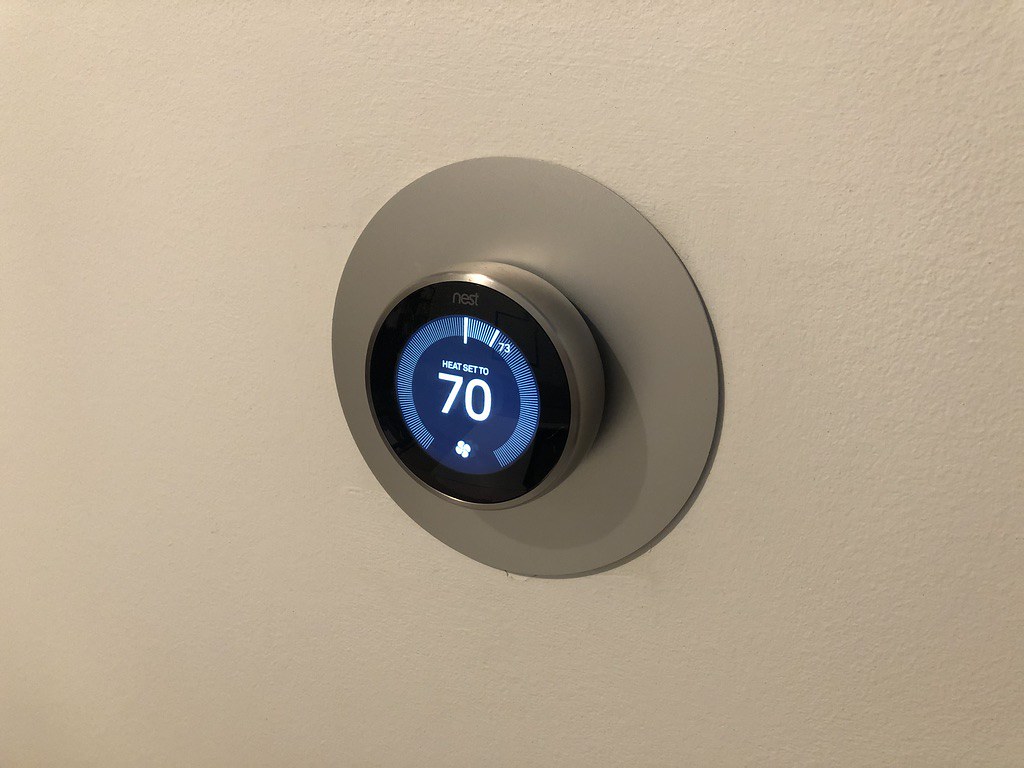This photograph captures a detailed wall-mounted thermostat set against a cream-colored plastered wall, illuminated by indoor synthetic lighting. The focal point of the image is a centrally positioned, round, silver-colored thermostat. It features a black digital display dial framed by a blue circular interface segmented with white lines, resembling an analogue clock’s hour markers from 7 to 5. Within the interface lies a digital readout indicating "Heat set to 70°F", alongside a small four-leaf clover-like emblem. The wall itself displays textured plasterwork, with the top right corner showcasing the intricate details of the paint roller's strokes, while the bottom left corner appears slightly out of focus and smoother. The observed shadows towards the bottom right of the thermostat suggest the primary light source is situated above and to the left. This setup likely functions as a temperature control device for managing indoor climate.